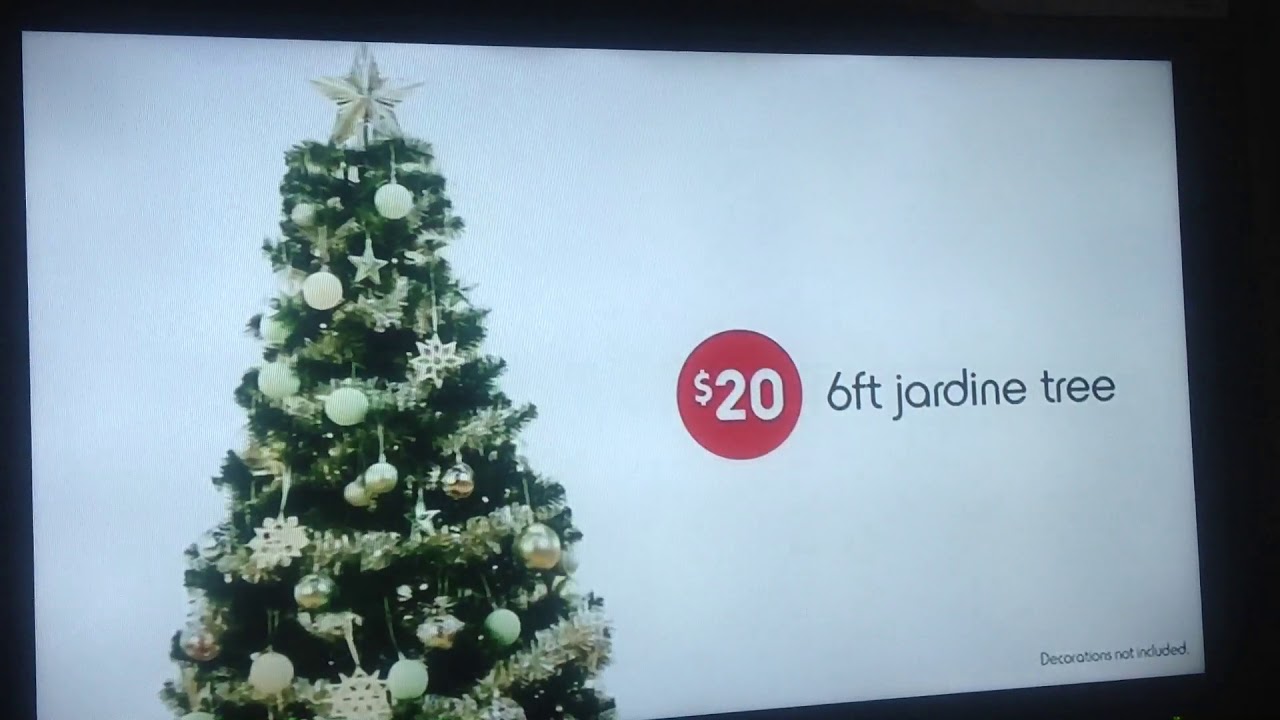The image features an advertisement displayed on a screen, promoting a Christmas tree. The background of the image is predominantly black, forming a narrow frame from the top to the bottom on the left side, similarly on the top, top to bottom on the right side, and on the bottom, it starts from the right-hand half, tapering towards the center. The screen itself has a light gray background. Centered on the screen is a dark green Christmas tree viewed from the front, adorned with numerous ornaments and topped with a gray star. To the right of the tree is a red circle containing the price "$20" in white text. Further to the right of the circle is text that reads "6-foot J-O-R-D-I-N-E tree." At the very bottom of the screen, in smaller text, it states "decorations not included," indicating that the ornaments seen are not part of the product offering. This detailed advertisement clearly highlights the tree and its price, ensuring customers understand what is being sold.